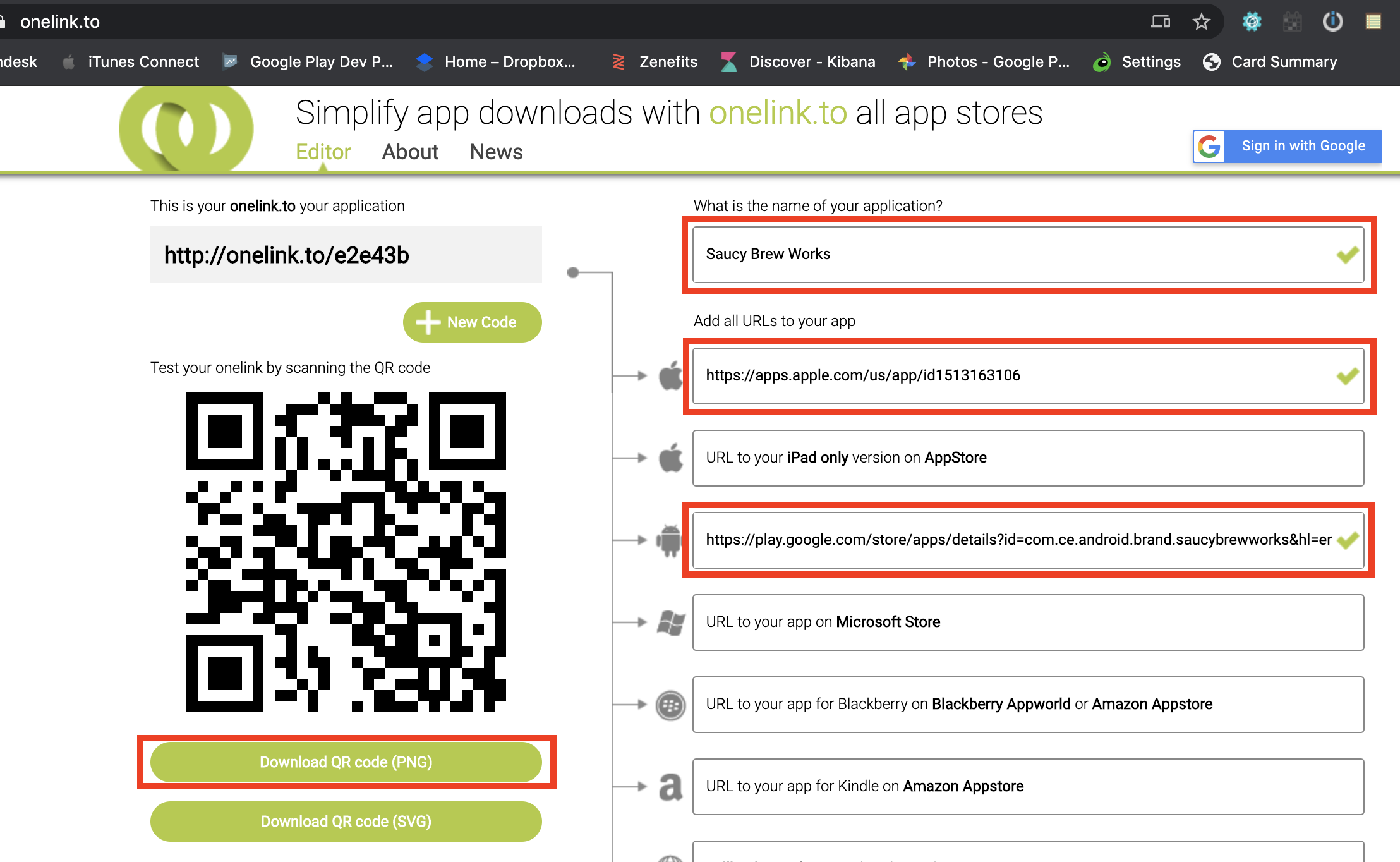A detailed caption for the described image could be:

"The webpage shown allows users to generate QR codes linking to various app store destinations using the onelink.to service. The interface lets you input the name of your application and URLs for different platform versions, such as iOS, iPad-specific destinations, and other relevant links. This setup is particularly useful for managing cross-platform downloads. The main feature on the page is the visual tool for creating and downloading these QR codes. Additionally, the user's workspace is personalized with bookmarks to frequently used services like Photos, Dropbox, and Google Play Store, but the focal point remains the QR code generation tool for streamlining app downloads."